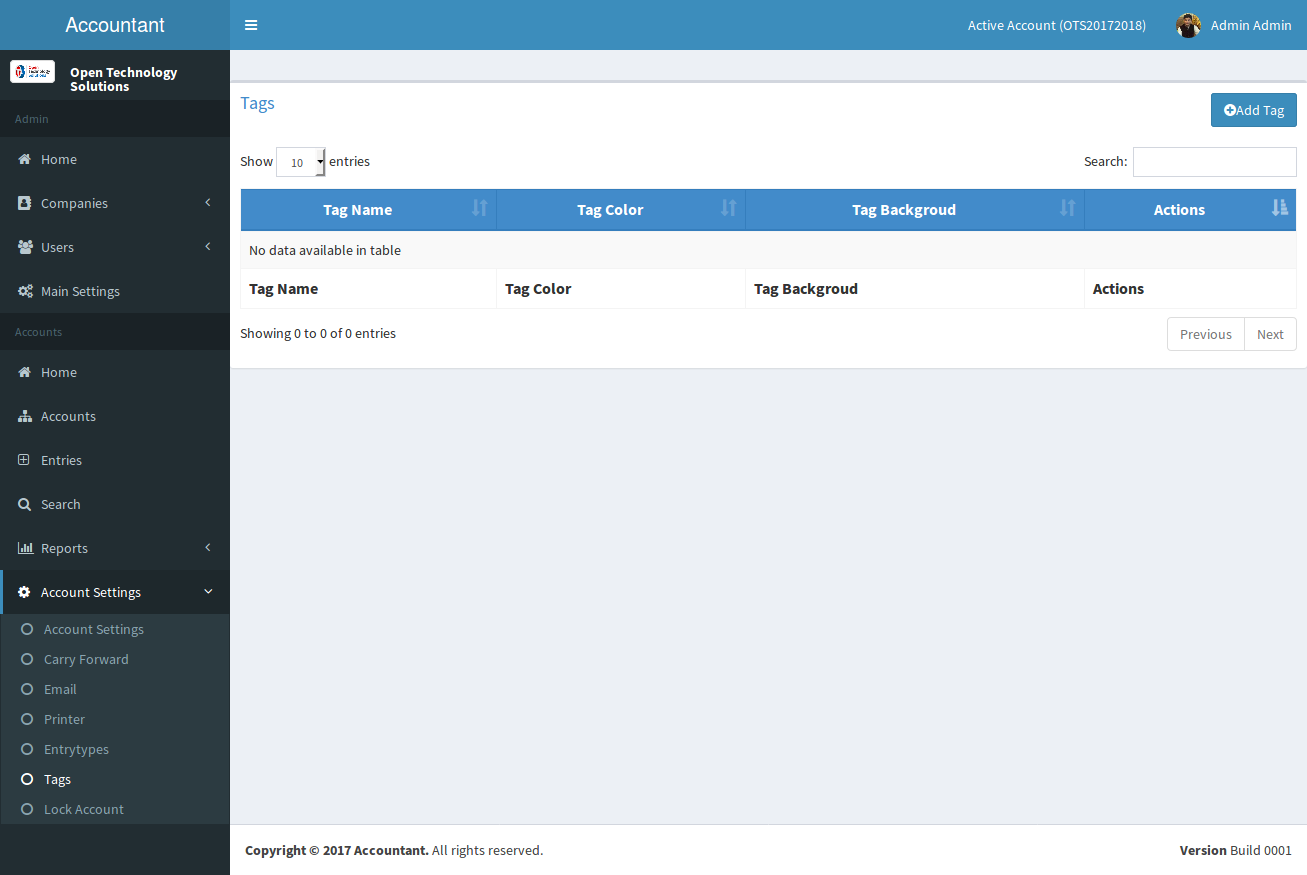Screenshot of the "Accountant" Program Interface:

At the top of the page, there's a prominent blue banner running horizontally. In the top-left corner of the banner, the text "Accountant" is displayed. To the right, there are three horizontal bars, indicating menu options. On the upper right-hand side of the banner, "Active Account (OTS 201 72018)" is written in white text. Beside this, a round profile picture is placed with the text "Admin, Admin" next to it.

The main content area features a white box centered towards the top, labeled "Tags." This box includes an option to add a tag, a line for "show entries," and a search bar. Below this box, another horizontal blue banner provides column headings: "Tag Name," "Tag Color," "Tag Background," and "Actions." Directly beneath this, in white text, the phrase "No data available in table" is displayed, indicating the absence of data entries.

Further down, the table headers are reiterated: "Tag Name," "Tag Color," "Tag Background," and "Actions," followed by the text "Showing 0 to 0 of 0 entries" indicating that there are currently no entries listed in the table.

The background of the page beyond this section is gray. On the left-hand side, a black and gray vertical bar runs down the page, containing additional menu options. At the top of this vertical bar, the text "Open Technology Solutions" is displayed.